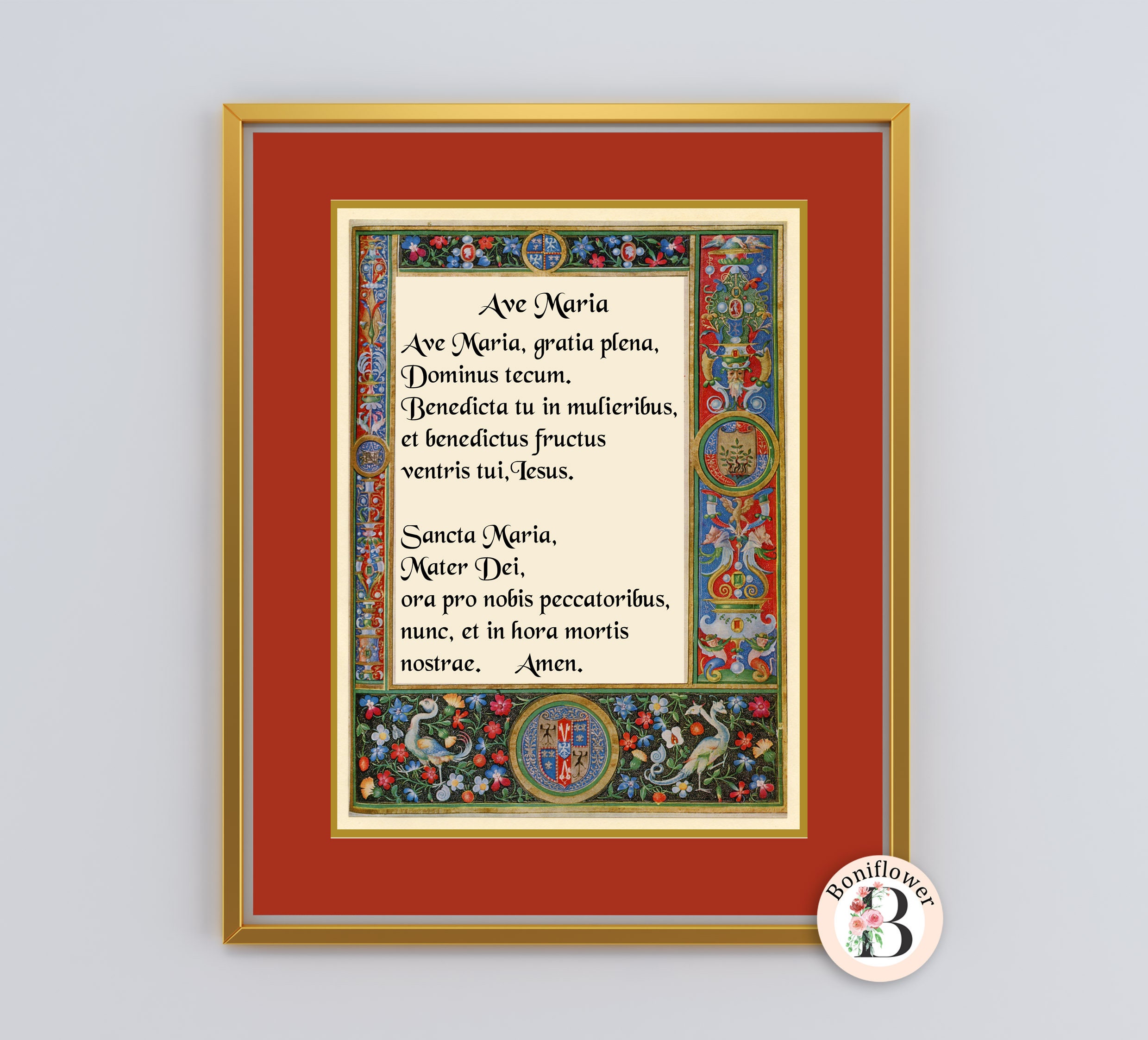This photograph captures an intricately framed artwork, possibly displayed in a museum or gallery, titled "Ave Maria." The centerpiece of the artwork is a text passage in Latin, beginning with "Ave Maria, Ave Maria Gratia Plana" and concluding with "Amen," suggesting a religious theme, likely a prayer. The text is encased within a rectangular field, richly adorned with red and blue floral designs, complete with green vines. Prominently in the center of the frame, a gold circle encloses a shield crest. Along the bottom, two chimera-like birds flank either side, adding to the regal and ornate aesthetic. The outer frame is predominantly red, lending a striking contrast to the detailed and colorful floral border and the central gold elements. Despite its realistic appearance, there is speculation that this piece could be a digitally edited artwork, potentially labeled "Bonnyflower B," featuring digital enhancements overlaying the frame, giving it an appearance that straddles between physical and digital art.